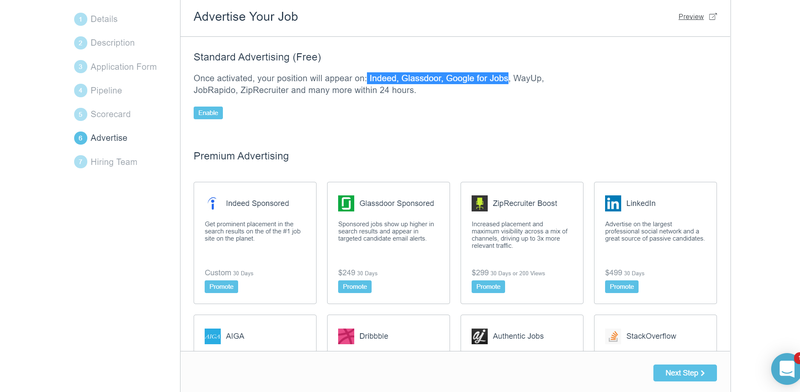This image is a screenshot of a job posting setup on Human Resource (HR) software, against a white background. 

On the left side of the screen, there is a vertical navigation panel featuring several labeled and numbered tabs: Details (1), Description, Application Form, Pipeline, Scorecard, Advertise, and Hiring Team. Each tab is accompanied by a corresponding blue circle with its respective number.

At the top center of the main content area, the heading "Advertise your job" is displayed in bold black font. Adjacent to this heading on the far right, there is a small underlined preview option in gray font, with a tiny share icon beside it.

Beneath the advertisement heading, the phrase "Standard advertising (free)" appears in bold gray font, followed by the text explaining that once activated, the job position will be visible on platforms such as Indeed, Glassdoor, Google for Jobs, WayUp, ZipRecruiter, and many more within 24 hours. The words "Indeed," "Glassdoor," and "Google for Jobs" are specifically highlighted within a blue bar. Below this information, there is a prominent blue button located towards the center-left.

Further down, a section titled "Premium advertising" is written in small black letters. Within this section, there are several small square boxes, each representing different recruiting websites. Each box contains the name of the website at the top, a short description under the name, and a button at the bottom to continue. These boxes are organized into horizontal rows of four.

At the bottom right corner of the screen, there is a blue "Next Step" button, ready to advance to the subsequent stage of the job posting process.